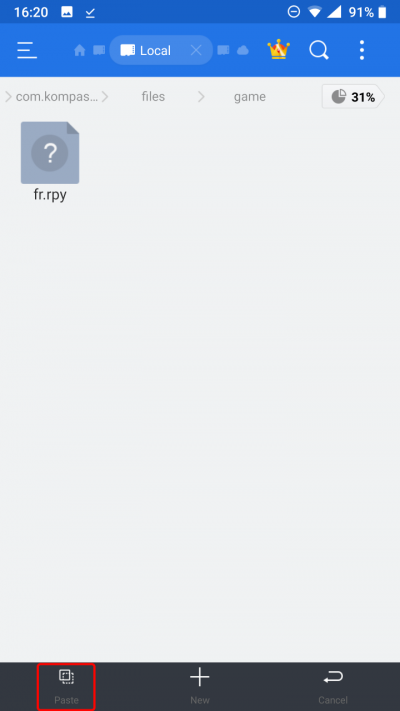In this image, we observe a screenshot with the timestamp "16:20" displayed in the top left corner. The phone's battery is at 91%, shown in the top right corner. Below the timestamp and battery icon, there is a blue navigation bar with a search bar labeled "Local." On the right side of this bar, there are three icons: a crown, a magnifying glass (search), and a three-dot menu.

The main content of the screenshot shows a directory path that reads "com.compass/files/game." Within this directory, there is a circular pie chart visual indicating 31%. The focus of the screenshot is on a gray file icon with a white question mark inside, titled "fr.rpy."

At the bottom of the screen, there's a dark gray bar with three buttons. The button on the far left, "Paste," is highlighted with a red outline. Next to it is the "New" button in the center, and the far right button is labeled "Cancel."